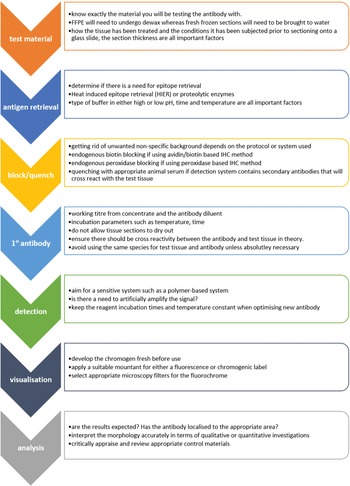The image is a detailed, digitally created flowchart likely designed for a science textbook, illustrating a step-by-step process with multicolored, downward-pointing arrows on the left-hand side. Each arrow is distinctively colored: orange, blue, yellow, light blue, green, black, and gray. The arrows are labeled sequentially with white text indicating various stages of a scientific protocol: "Test Material," "Antigen Retrieval," "Block/Quench," "Primary Antibody," "Detection," "Visualization," and "Analysis." 

To the right of each arrow, there is a corresponding text box bordered in the same color as the arrow. Though the text within these boxes is too small to read clearly in the provided details, it is implied that each box contains a few sentences or bullet points describing the specific activities or considerations relevant to each stage. For instance, the "Test Material" box likely discusses different preparation methods for various types of samples, while subsequent boxes delve into specifics such as epitope retrieval methods in the "Antigen Retrieval" stage, and the importance of section thickness. This structured and comprehensive chart serves to guide users through the procedural steps necessary for preparing and analyzing a specimen, making it a valuable educational tool in scientific studies.